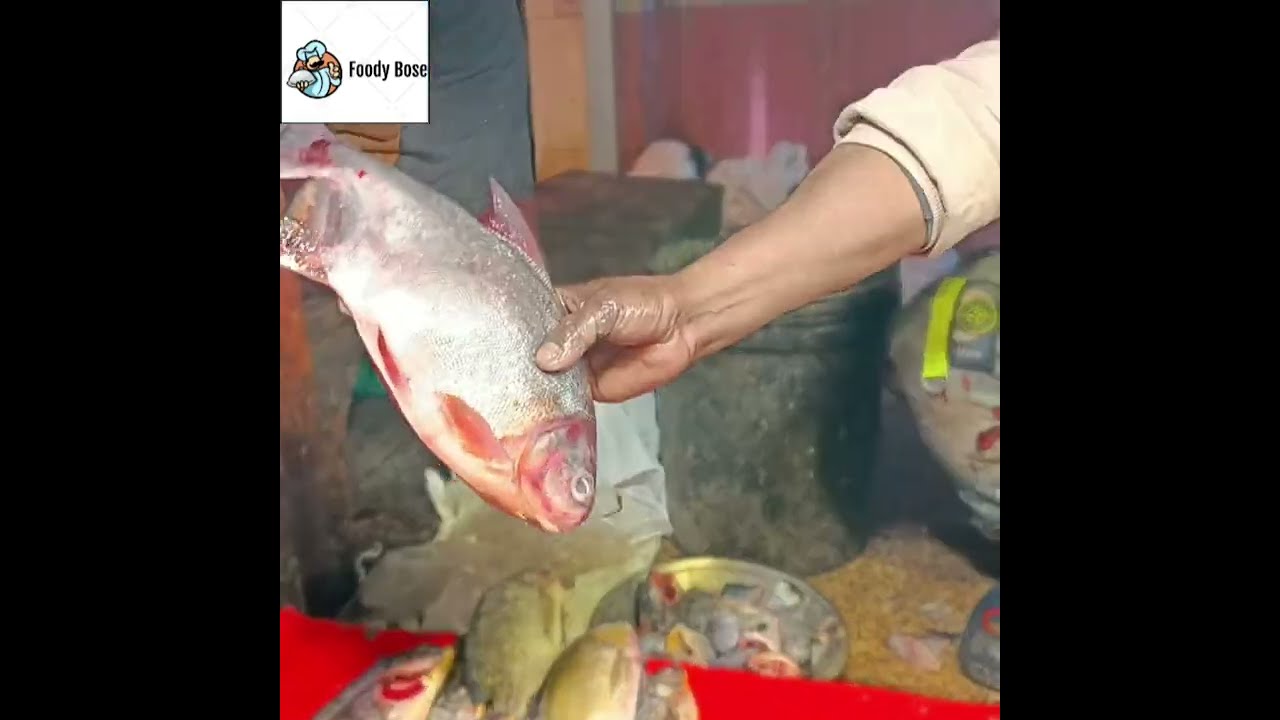In this image, we can see a bustling, possibly worn-out fish market setting. At the forefront, a man's hand extends from the upper right corner, clad in a rolled-up white long-sleeve shirt, grasping a plump, shiny silver fish with striking red fins and a red-tinged head, evoking a slightly bloody appearance. This fish is held prominently towards the camera, with the man's thumb clearly visible. Below the hand, a red table, perhaps covered with a red tablecloth, is heaped with similarly sized and colored silver-yellow fish, neatly stacked. The scene is further enriched with the background showing old steel buckets brimming with various fish, enhancing the market atmosphere. Additionally, in the upper left corner, a small logo featuring a chef holding a platter is visible with the inscription "Foodie B.O.S.E." indicating a possible branding or thematic element. The overall image is enclosed with black borders on the left and right sides, giving it a framed appearance.